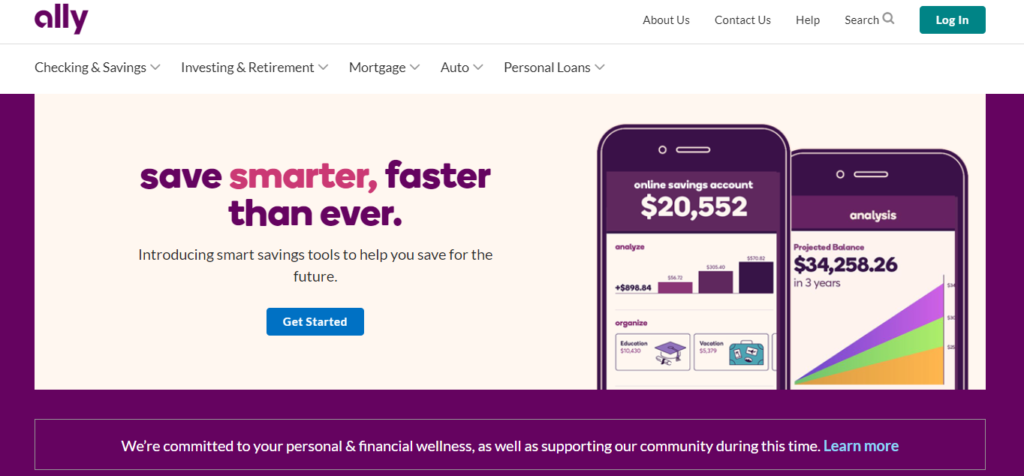A detailed full-color screenshot of a financial services website. In the top left corner, "ALLY" is prominently displayed in deep purple. On the top right, there are navigation options including "About Us," "Contact Us," "Help," a "Search" bar, and a "Login" button on a green background.

A thin, narrow grey line separates the header from the main content. Below this line, on the left, is a menu listing services: "Checking and Savings," "Investing and Retirement," "Mortgage," "Auto," and "Personal Loans," indicating that they are a financial services company. A purple band frames the bottom and sides of the page, with the following text at the bottom: "We are committed to your personal and financial wellness, as well as supporting our community during this time." A "Learn more" link is highlighted in blue.

A cream rectangle dominates the main section, featuring text on the left: "Save" in purple, "Smarter" in pink, and "Faster Than Ever" in purple. The caption reads, "Introducing smart savings tools to help you save for the future," accompanied by a blue "Get Started" button. On the right side of this rectangle, there is an image of two mobile devices, with the left device slightly higher and overlapping the right one. Both devices have black bands at the top, followed by purple bands.

The screen on the left device displays a savings account with a balance of $20,552 and a small graph showing three different saving lines below. Further icons are partially visible. The right device illustrates an "Analysis" with a balance of $24,258.26, featuring a triangular graph colored orange at the bottom, green in the middle, and purple at the top, indicating a trend from the lower left to upper right.